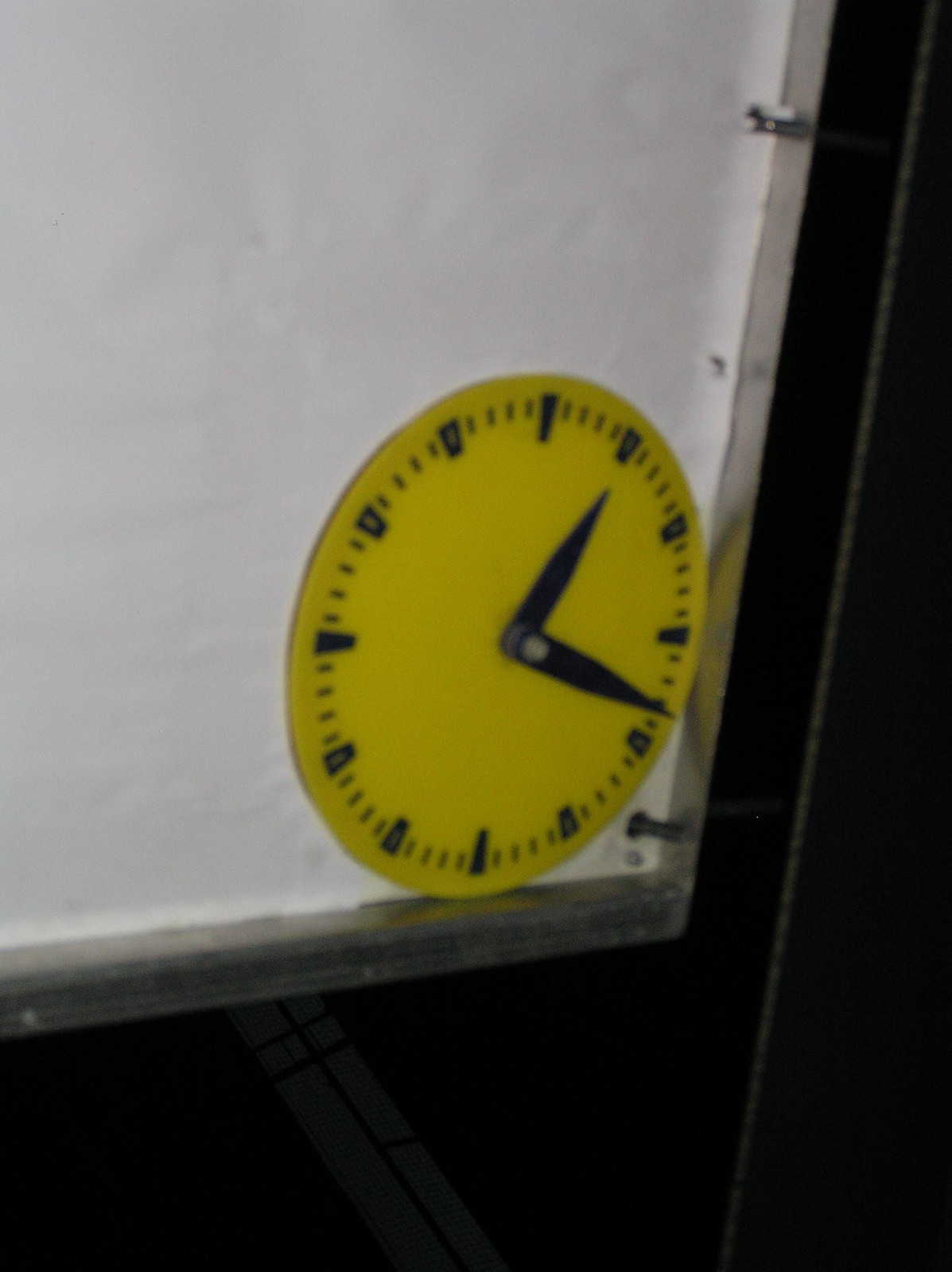This photograph showcases a minimalist yellow flat plastic clock positioned in the window section of a door. The clock is notable for its simplicity, featuring black hands indicating the time as 1:18. Absent of numerical markers, the clock face displays thick lines to denote the hours and four thin lines between each for the minutes. The clock is framed by a silver metal border set within the door's window cut-out, which is covered by a white paper-like material instead of glass. Surrounding this window, the scene transitions into a dark backdrop with white baseboards visible along the bottom edge. Additionally, a white diagonal line stretches from the top right corner to the bottom, cutting through the dark background and adding an intriguing visual element to the composition.